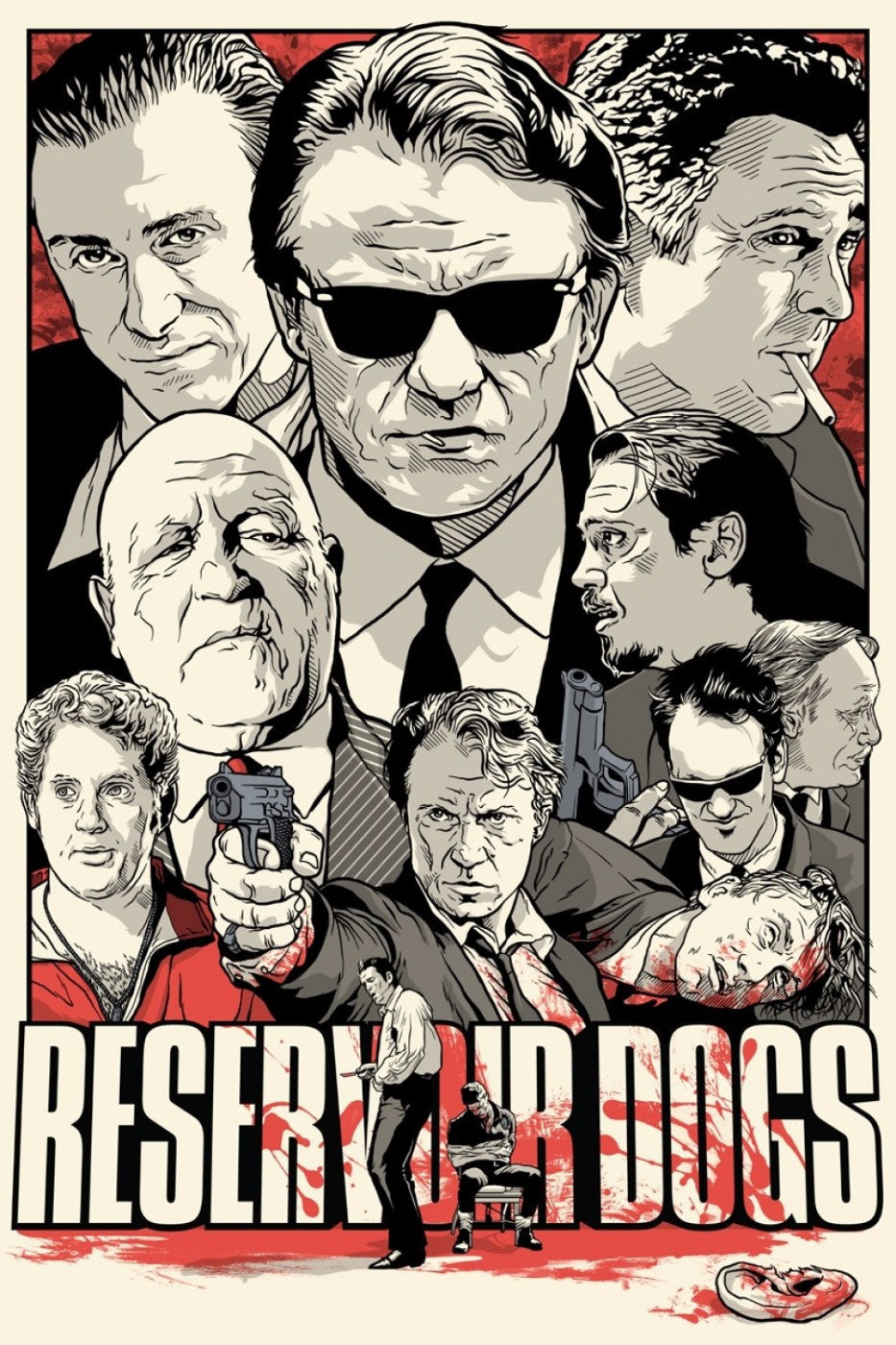The poster is a pop art-style depiction of the film "Reservoir Dogs," rendered in a sketch manner reminiscent of Grand Theft Auto aesthetics. The majority of the movie's dominant characters are featured, totaling ten. The artwork is mostly in black and white with strategic splashes of red. In the lower part of the poster, a man tied to a chair is confronted by another man standing in front of him with his back turned. The title "Reservoir Dogs" is displayed at the bottom in white letters, accented with blood splatters. Above this intense scene, larger headshots of eight characters dominate the composition. These characters all share serious, determined expressions, with details such as sunglasses, toothpicks, and cigarettes contributing to their cool, menacing look. Notably, one man at the center with a suit, toothpick, and sunglasses stands out, flanked by two others, one holding a cigarette. Additionally, a man in the bottom center aims a gun, adorned with a red splash, while another character appears dead, adding to the dramatic and violent atmosphere.